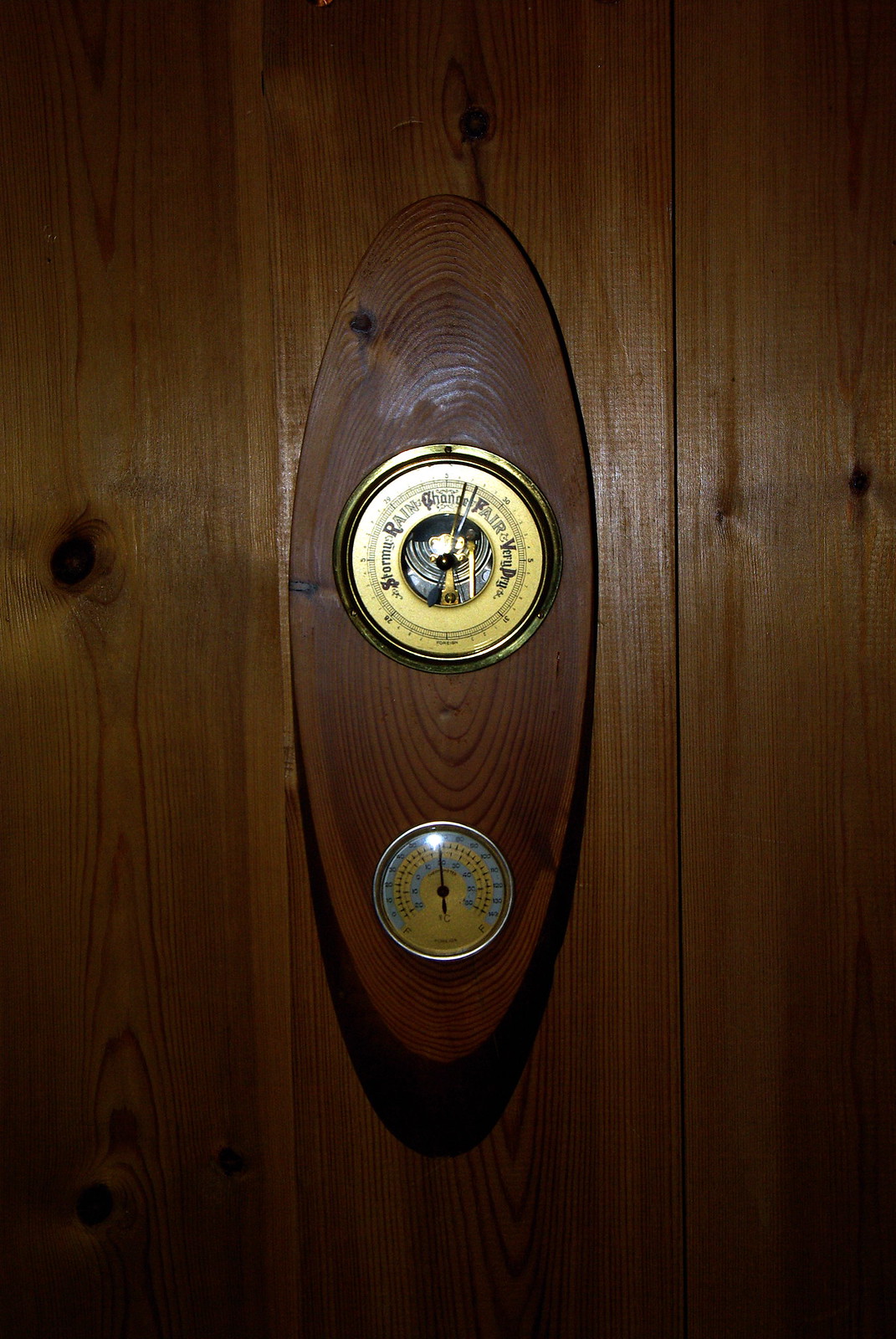The image displays a close-up of an intricately detailed object mounted on a dark brown-paneled wooden wall, which bears black spots suggestive of aged paneling. The wall appears to consist of three visible panels with subtle hints of dark brown and green tones. 

Central to the image is an oval-shaped, vertically oriented object, darker in hue than the wall, showcasing a pronounced wood grain pattern with approximately 50 rings. Dominating the center of this oval are two distinct circular elements. 

The upper circle, positioned nearly at the center, features a gold rim and interior, encasing a delicate gold needle. This element resembles a clock but is adorned with elaborate inscriptions and symbols, possibly indicating it is measuring other variables. The interior workings of this circle, visible through the gold encasement, reveal components that are blue or silver in color.

Beneath this, the lower circle is trimmed with a silver rim and has a yellow and white interior. It houses a needle, either white or black, suggesting it could be a temperature gauge or another type of measuring instrument.